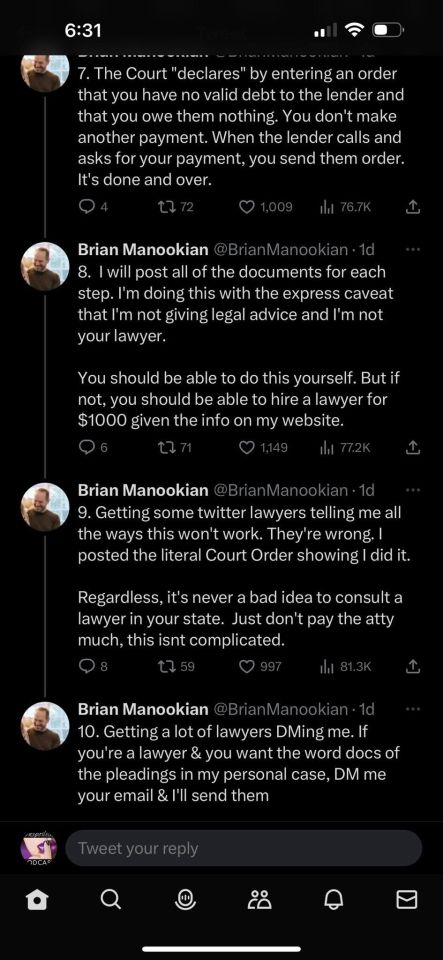Here is a cleaned-up and detailed descriptive caption for the provided image:

---

The screenshot is taken from a device with dark mode activated, featuring a black background and white text. The status bar at the top displays the time as 6:31, with indicators showing full WiFi connectivity, several cell phone signal bars, and approximately half battery life remaining. 

The main content consists of four images of a man, who appears to be in his mid-30s, with a light complexion, looking to the left. He is wearing a grayish-green shirt. Surrounding these images is a considerable amount of text, predominantly in white font.

In the text, the author discusses a court order that declares the individual has no valid debt to a lender and should not make any further payments. They mention that, upon receiving a payment request, the individual should send the court order to the lender, effectively resolving the debt issue. The author offers to post the necessary documents for each step of this process but emphasizes that they are not providing legal advice. They suggest that while individuals can manage this process on their own, they have the option to hire a lawyer for approximately one thousand dollars, providing the lawyer with information from the author's website.

The author, identified as Brian McClooney, mentions that some have criticized the validity of the court order posted on social media platforms like Twitter, but insists that the order is legitimate. They offer to share Word documents related to this process with any interested lawyers and invite people to contact them directly via direct message (DM) for further details.

---

Note: While this enhances readability and ensures a structured layout, the exact phrasing of sensitive information can vary to ensure accuracy and appropriateness based on actual legal contexts.